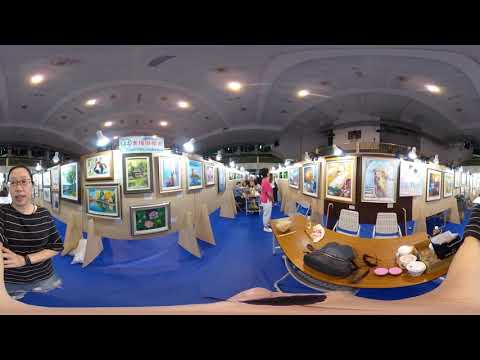This is a photograph of an indoor art gallery captured with a fisheye lens, creating a curved panoramic effect. Two fisheye views frame the image, showcasing a high-ceilinged room with gleaming white overhead lights. The cobalt blue floor contrasts with the tall white ceiling, which has arched windows at the back. The walls, painted green, are adorned with numerous colorful paintings, both vertically and horizontally framed, distributed in structured aisles that lend the space an orderly aesthetic.

In the foreground, there is a brown wood counter with a modern small cash register or sales device, flanked by two empty chairs. A woman standing beside the counter looks towards the camera; she is dressed in a black shirt with white horizontal stripes. On the left side of the image, an Asian man, also in a black t-shirt with white stripes, wearing light-rimmed glasses and a wristwatch, approaches the counter. The fisheye effect accentuates the curvature of the scene, making the aisle and surrounding walls appear to bend unnaturally, adding a unique visual dimension to the gallery space.